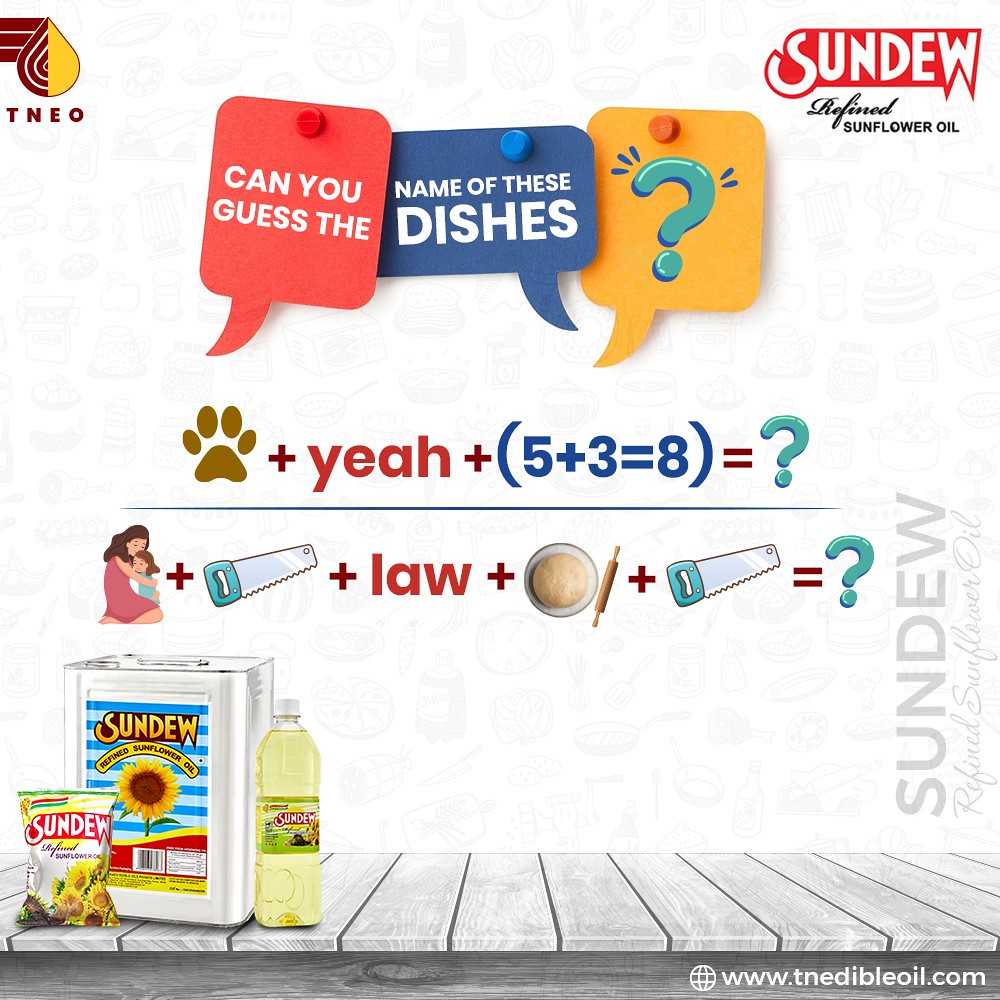The image is a vibrant, digitally created advertisement for Sandu refined sunflower oil, with various elements cohesively tied together. At the top right corner, in bold white lettering against a red background, it says "Sandu" and "sunflower oil." Below this, three colorful cardboard speech bubbles are pinned, with the phrases "Can You Guess The" in a red bubble, "Name of These Dishes" in a blue bubble, and a teal question mark in a yellow bubble.

Beneath the speech bubbles, there's a playful puzzle involving primary colors where a series of equations are depicted. The first part shows a paw print, a plus sign, the word “Yeah” in red, plus 5 plus 3 equals 8, ending with a teal question mark. Below a division line, there's a more intricate puzzle featuring a mother hugging her child, a plus sign, a saw, the word “law,” a plus sign, a loaf of bread and a rolling pin, another plus sign, another saw, all followed by a question mark.

At the bottom of the image, there are various containers of Sandu sunflower oil: a bottle of cooking oil, a large box-version of the product, and a package of chips, all adorned with the Sandu logo and sunflowers. The entire scene is set against what appears to be a deck, making for an inviting and eye-catching advertisement.